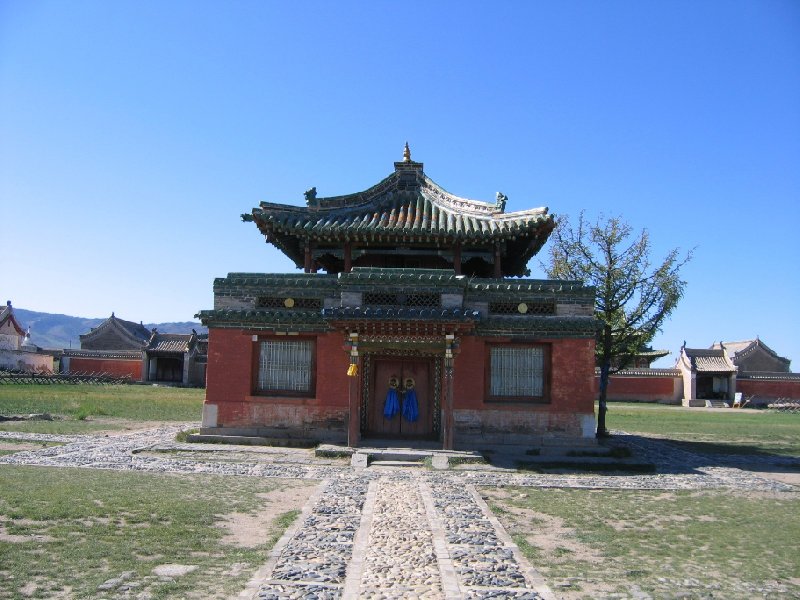This photograph captures a central building of Asian origin, featuring a prominent pagoda-style roof crafted from jade green terracotta tiles. The building's main body is constructed of red brick, accentuated by a pair of double doors with brass handles, adorned with silky blue streamers. Two windows flank the entrance, contributing to the building's balanced design. The hand-laid stone walkway encircles the building, bordered by a small tree to the right. The entire scene is set against a backdrop of a vivid blue sky without a cloud in sight. Surrounding the main building, additional structures of a similar architectural style create an impression of an ancient city or a complex of traditional buildings. The photograph, capturing an outdoor setting, hints at a sparse yet harmonious landscape featuring grass, dirt, and visible hills in the distance, offering a serene and picturesque view.